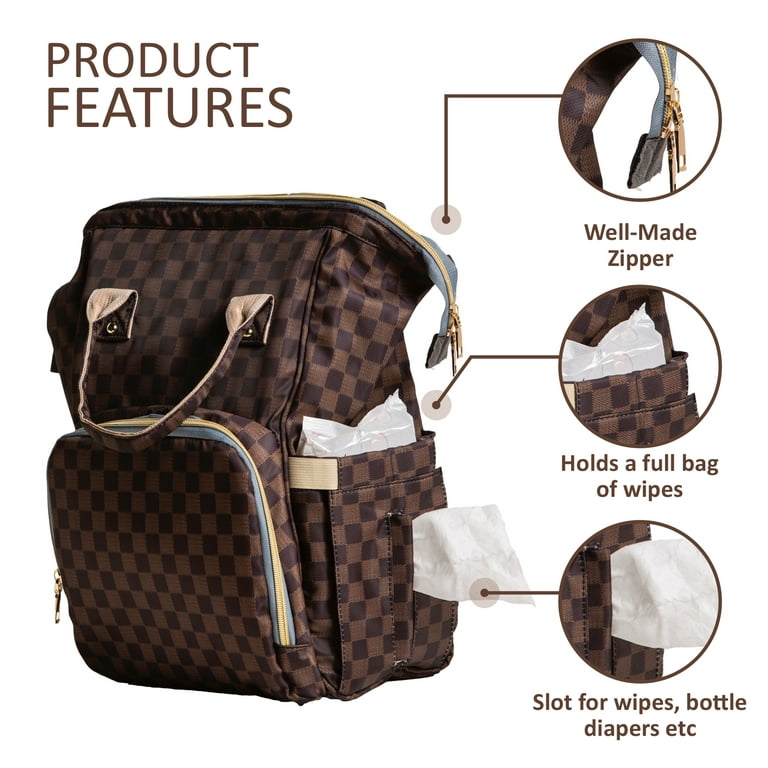The image showcases an advertisement for a checkered diaper bag styled as a backpack with a solid white background and no border. In the upper left corner, the words "PRODUCT FEATURES" are stacked vertically in all-cap, brown print. To the left of the text, there is a frontal and side view of the bag, which is adorned with a checkerboard pattern of alternating dark brown and medium brown squares. The bag features a light brown handle on the front and a gold zipper on a zippered pocket also located on the front side.

On the right side of the image, there are three vertically arranged circles emphasizing specific parts of the bag with close-up views. Each circle has a corresponding line pointing to a different feature on the bag. The first circle highlights a "well-made zipper," the second circle indicates it "holds a bag full of wipes," and the third circle points out a "slot for wipes, bottle, and diapers," showing a tissue extending from the slot. The bag appears to be constructed from a vinyl material and is designed with practicality in mind, presumably aimed at parents.